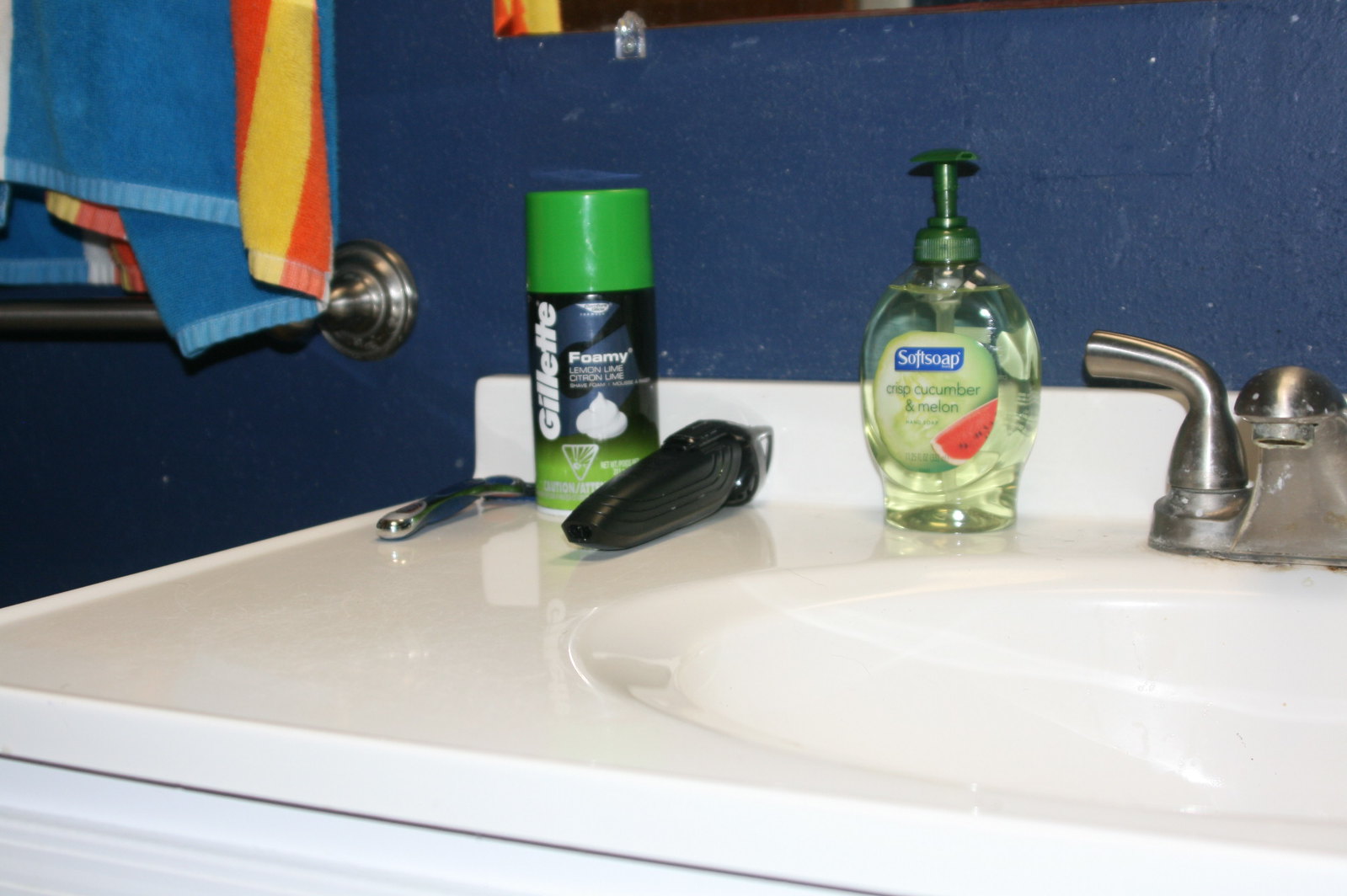A detailed and cleaned-up caption for the image could be:

"This image captures the interior of a bathroom sink area, viewed from the front. The sink, framed by a dark blue wall, features a silver metallic faucet with a single visible handle, bent and positioned to the left. The sink's surface holds various personal care items. On the left, there's a clear plastic bottle of hand soap with green liquid inside and a darker green dispenser. Beside it lies a black electric shaver. Adjacent to the shaver is a bottle of Gillette shaving foam, characterized by a black container with a green cap and base, adorned with a white foam graphic on its label. A silver-handled razor blade rests face down nearby. Above the sink, affixed to the wall, is a towel rack holding a vibrant blue towel with bright orange and yellow stripes along its edge."